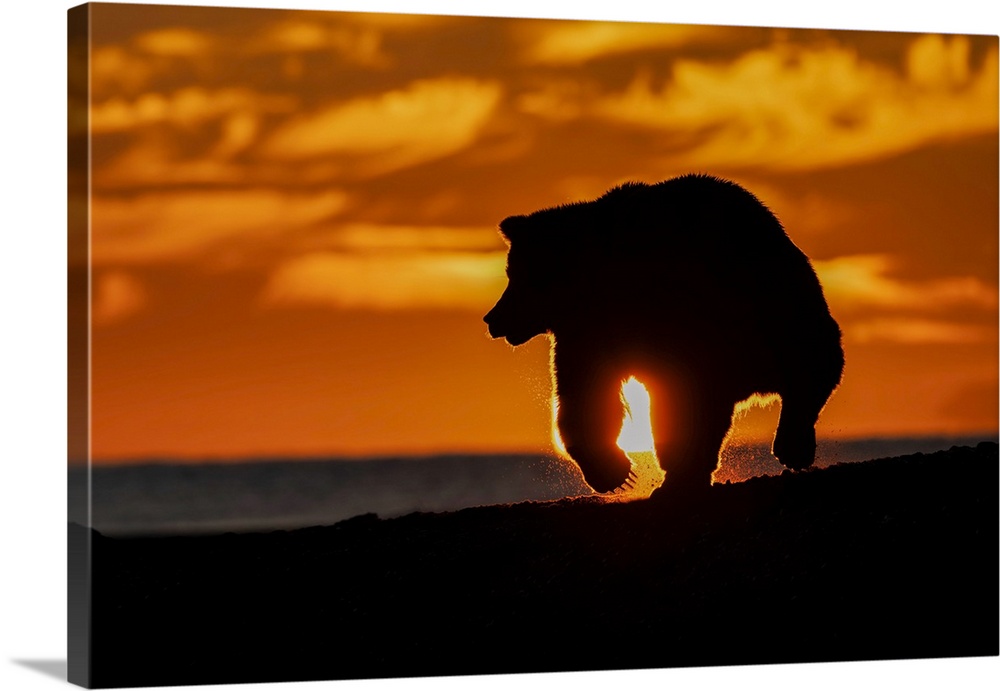This detailed nature canvas print captures the dramatic silhouette of a large bear walking along a beach at sunset. The rectangular print, oriented in landscape view, features the bear facing left, its front right paw slightly lifted revealing sharp claws. The golden sky, interspersed with clouds, creates a stunning backdrop, while the blurred grayish-blue ocean can be seen just above the dark, almost black, beach. The setting sun, positioned directly behind the bear, peeks through its legs, casting a shadow and highlighting the bear's outline, ears, nose, and mouth. The bear's fur texture and long claws are visible against the deepening evening light. Notably, the textured canvas adds a three-dimensional effect, with a slight shadow cast on the wall behind it on the left. This blend of vivid and muted colors, alongside the interplay of light and shadow, creates a captivating and serene moment in nature.